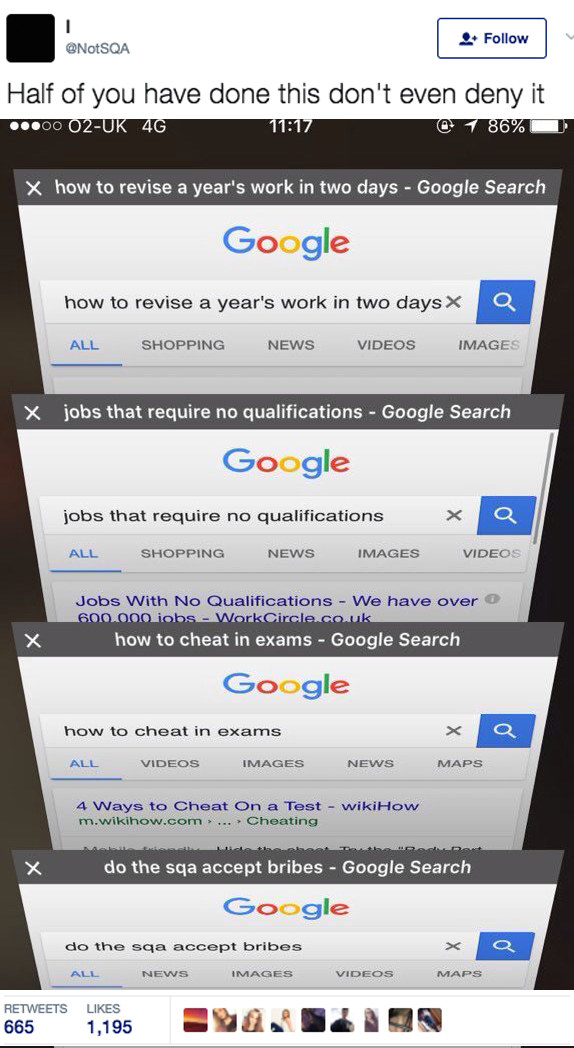This screenshot, captured from a mobile device, displays a humorous post on a social media platform created by a user named @notSQA. The image is a composite showing four stacked Google search results that mockingly illustrate the frantic online searches of a desperate student. The searches include: "how to revise a year's work in two days," "jobs that require no qualifications," "how to cheat in exams," and "do the SQA accept bribes." At the top, in bold black text, the caption reads, "Half of you have done this, don't even deny it," suggesting a relatable yet exaggerated scenario. In the top-right corner, there’s a follow button, indicating the user’s profile can be followed. At the bottom of the screenshot, near the navigation bar, the statistics show the post has received 665 retweets and 1,195 likes. Additionally, there are nine user icons in different colors, likely representing those who have engaged with the post. This cleverly composed image pokes fun at the lengths students might go to during exam season.